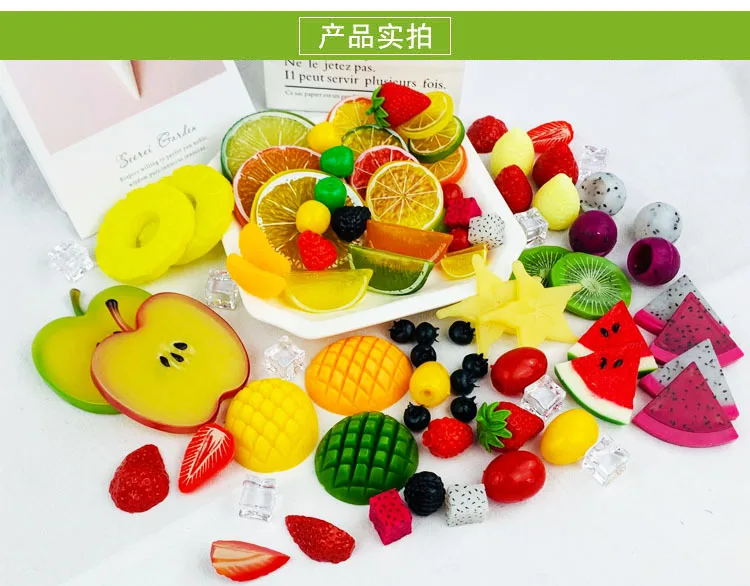The image displays a variety of vividly colored plastic fruit, meticulously arranged on a white tabletop. The assortment includes slices and wedges of watermelon, kiwi, apples, pears, pineapples, oranges, strawberries, blackberries, raspberries, lemons, limes, mango, dragon fruit, blueberries, and even tomatoes. Some of the fruit pieces are notably shiny, giving them a plasticky appearance. There are also small, clear, plastic ice cubes scattered among the fruit. In the center of this display, a small plate is positioned. Above the array of fake fruit, a green rectangular strip with four Japanese characters in a small white box is visible, suggesting a Japanese origin. Additionally, there are paper signs protruding from the top edge of the image, one of which contains French text, further highlighting the international aspect of the display.